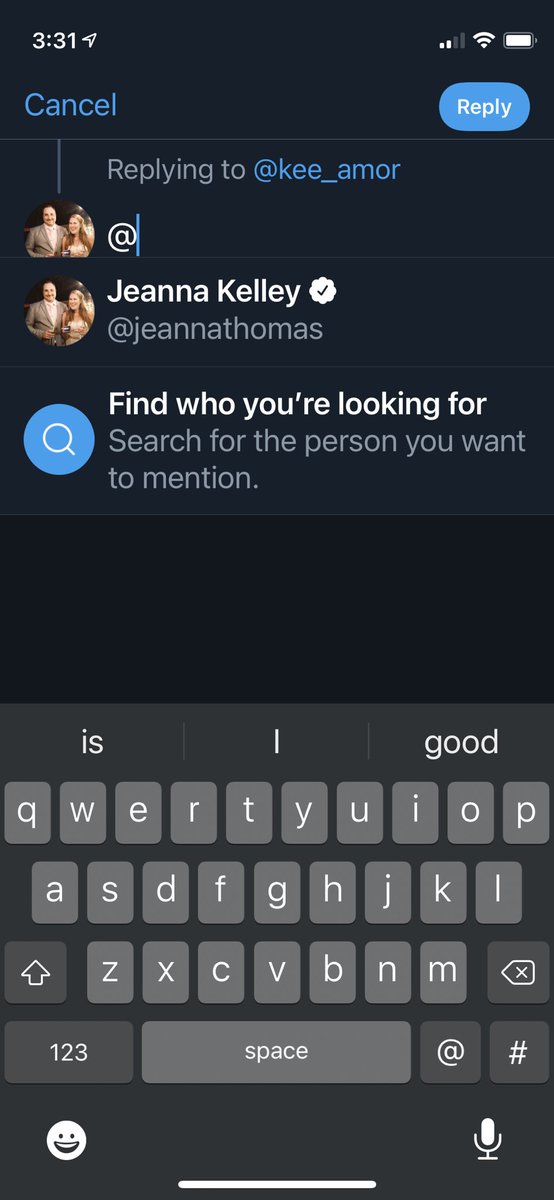This image is a detailed screenshot from a mobile device in dark mode. The device's status bar at the top right features standard indicators: a battery icon, Wi-Fi signal strength, and cell signal strength. The time displayed in the upper left corner reads 3:31, accompanied by an arrow icon indicating active location services. The screenshot captures a section of the Twitter app, highlighting a reply interface.

In the app, a header text reads "Replying to @key_amour." Directly below this, there's a small circular profile picture of a couple, appearing to be white, though the image is not clear due to its small size. Next to the profile picture is a cursor, visible as a blue vertical bar, indicating the area where the user can type their reply.

Further down, the Twitter user ‘Gina Kelly’ is detailed, with her name uniquely spelled as "G-E-J-E-A-N-N-A-K-E-L-L-E-Y". She has a white check mark (likely indicating a verified account), and her handle is @GinaThomas.

At the bottom of the screenshot, the device's onscreen keyboard is visible, indicating that the user is in the process of typing a reply tweet.